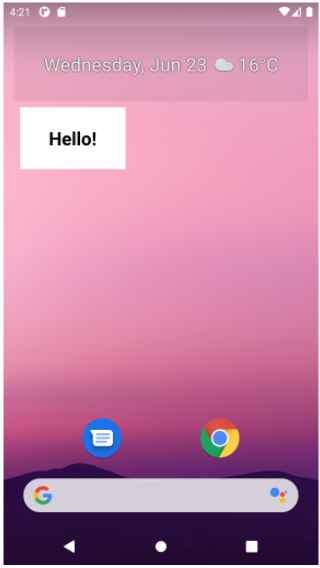Screenshot of a smartphone's home screen showing: 

- **Status Bar**: Displays the time "4:21" alongside a circle and a square icon. To the right, Wi-Fi signal strength is indicated by a "pie piece" icon, network signal strength by a triangle with three or four bars, and a fully charged battery icon.
- **Background**: A serene sunset featuring light pink hues at the top transitioning to maroon at the bottom. The silhouette of mountains is prominently visible at the bottom edge.
- **Top Status Information**: The date "Wednesday, June 23rd" is accompanied by a cloud icon and the temperature "16°C."
- **Main Section**: A large white square with the text "Hello!" followed by an exclamation point.
- **Bottom Section**: 
  - Icon representations of the Text Messaging app and the Google app near the mountain silhouette.
  - A Google search bar featuring a 'G' on the left appears just below the app icons.
  - Navigation bar containing a triangle (Back), a circle (Home), and a square (App Switcher) icon at the very bottom.